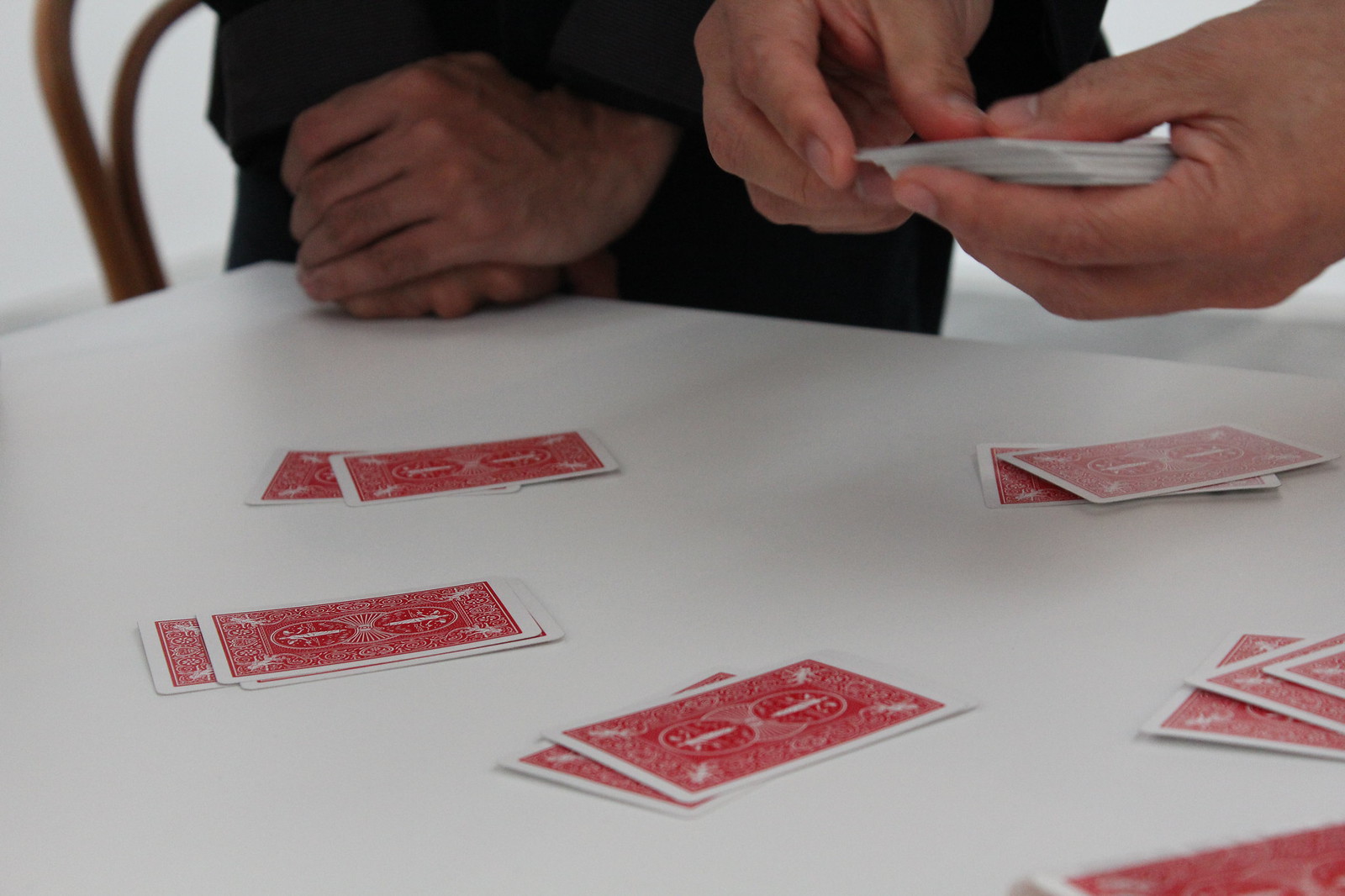A detailed close-up image captures two hands engaged in a card game on a white table surface. The first pair of hands, belonging to an individual dressed in a black long-sleeved shirt, are folded and resting calmly on the table. The second pair of hands is actively shuffling a deck of cards. On the table, six neatly arranged stacks of cards are visible, each stack consisting of two cards placed one on top of the other, all face down. The backs of the cards display a red and white pattern, adding a touch of color to the otherwise monochromatic scene.